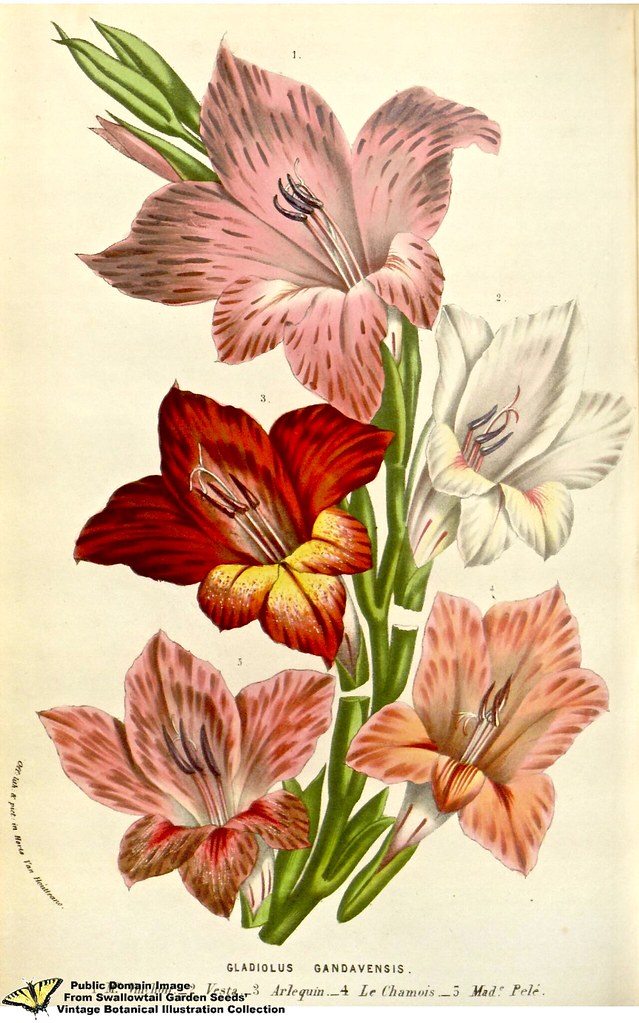The image portrays a vintage botanical illustration, featuring a tall art print with an aged, pale yellow background. Centered on the poster is a single green stem that extends from the bottom to the top, curving gently to the upper left and displaying five distinct blooms along its length. Each flower, sharing the same species, exhibits unique colors and gradations. 

At the top, the largest bloom showcases a pale pink, almost salmon color with darker brown striations. Below it, on the left, a dark red flower with yellow and orange overtones stands out, its stamen prominently dark. To the right, a nearly albino white flower has faint red tones central to its petals. At the bottom, two similar pink rosé flowers with darker red striations can be seen; the left one features a dark stamen, while the one on the right has a much lighter stamen.

Captioned in black at the bottom left of the image, the text reads "Public domain image from Swallowtail Garden Seeds, vintage botanical illustration collection," accompanied by a small yellow butterfly. The central bottom text, also in black, identifies the species as "Gladiolus gandivinensis," followed by the names "Vesta, Arlequin, La Camoisse," with additional curved text that's hard to read.